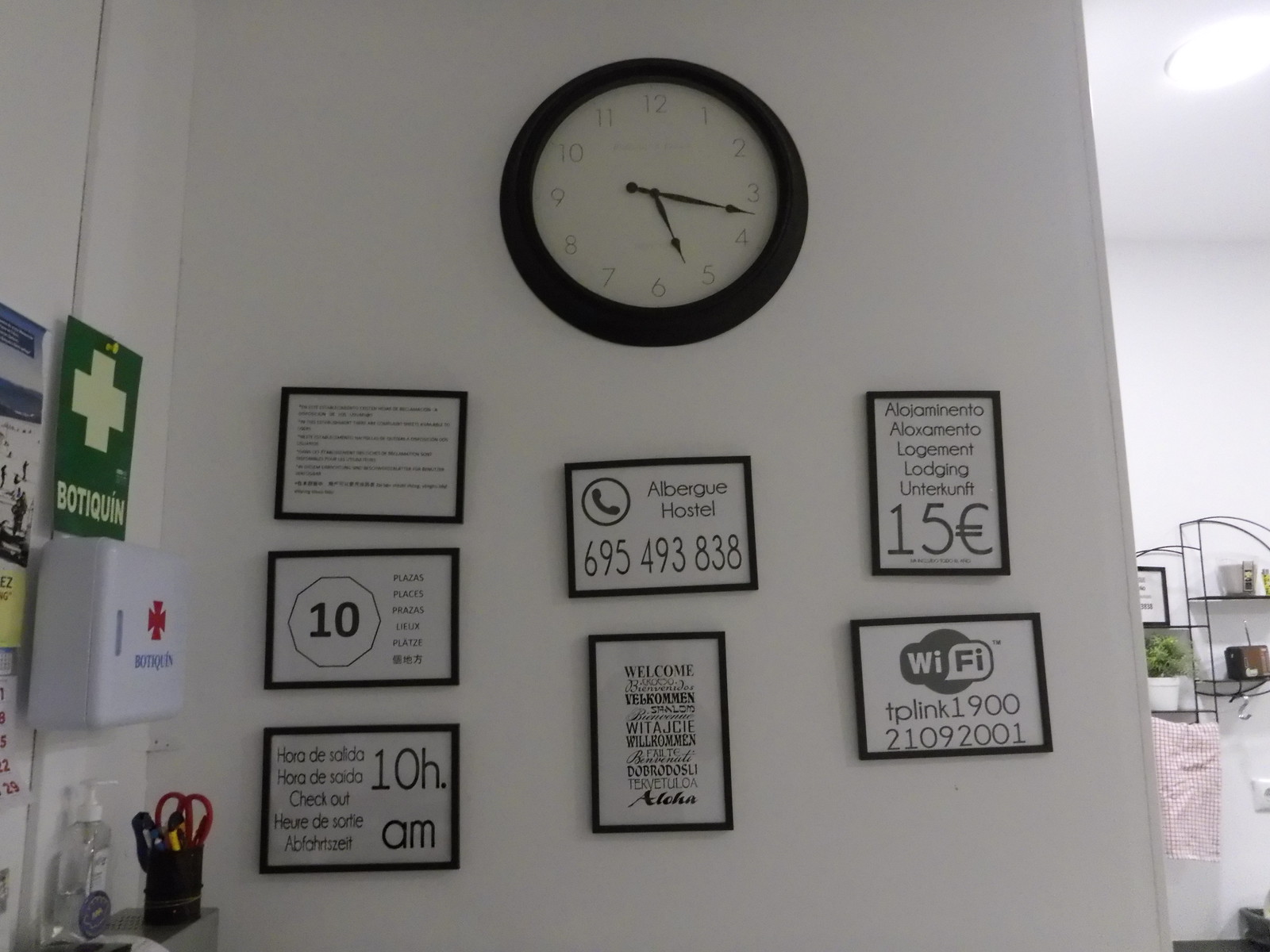This photograph captures a minimalist, predominantly white wall with various elements arranged against it. Centered at the top of the wall is a round clock, featuring a white face encased in thick, black framing. The clock displays the time as 5:17, with its numerals in light black and the hour and minute hands in a darker black for contrast.

Beneath the clock, three vertical rows of framed pictures are symmetrically aligned next to each other. Each frame is black, enclosing a white background adorned with black writing, creating a cohesive monochromatic aesthetic.

On the left side of the image, the corner of the wall is visible, with an adjacent wall extending from it. Mounted on this secondary wall is a white first aid box. Directly above the first aid box is a green square sign, prominently featuring a thick, light green cross. Beneath this cross, white writing is clearly displayed, indicating its purpose or instructions related to the first aid emergency kit below.